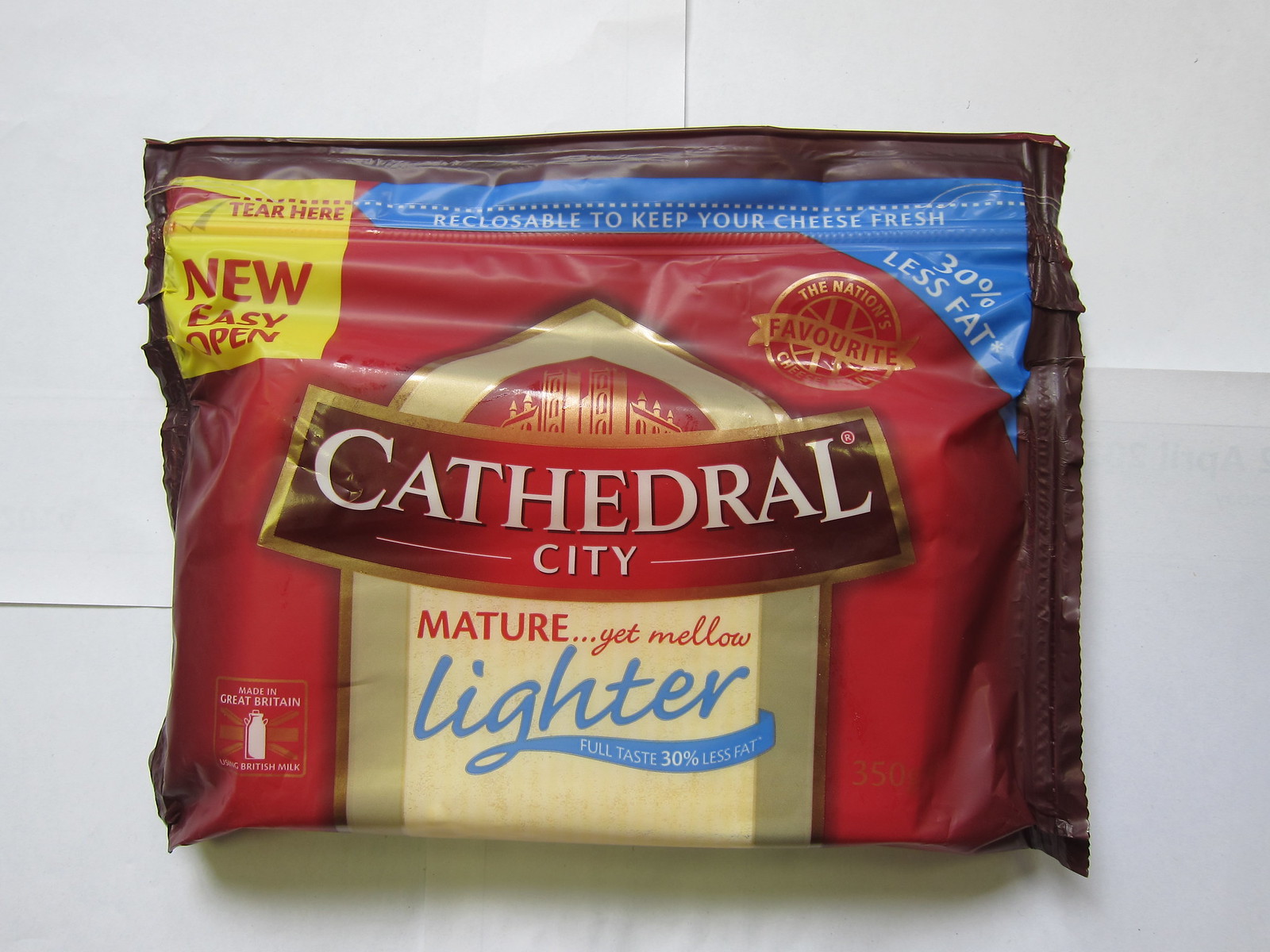The photograph features a package of cheese on a white background. The package, which has a ziplock seal, is predominantly red with a yellow square at the top left corner that says "Tear Here" and "New Easy Open" in bold red text. Below this, there’s a yellow triangle on the top right corner that reads "30% Less Fat." A blue banner across the top states, "Re-closable to keep your cheese fresh." In the center, the package displays a logo resembling a cathedral with a red-topped structure, and underneath it in a curved red banner with white print, it reads "Cathedral City." Below this, there's a yellow background with the words "Mature... yet mellow" in red text and "Lighter" in blue cursive. Additionally, the package notes "Made in Great Britain" at the bottom left corner.